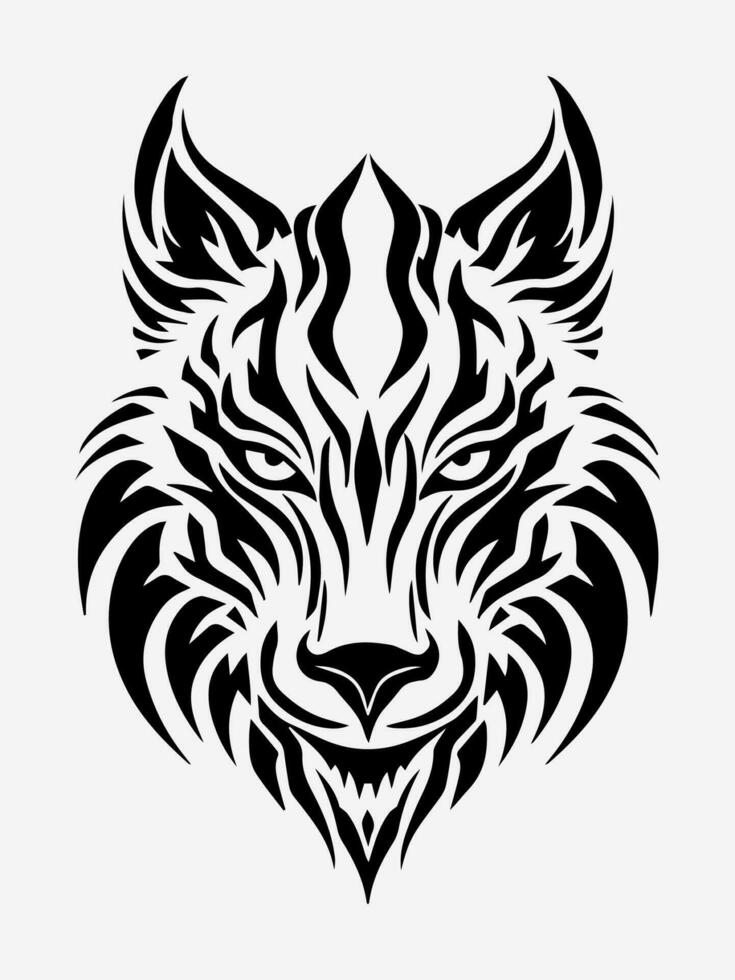This detailed black and white image, likely a design meant for a tattoo, intricately depicts the front view of a wolf with a heavy tribal influence. The design features a stark contrast with a white background, utilizing bold, black lines to shape the animal. Its black ears curve gracefully upward and toward the center, framing the composition. The wolf's eyes are depicted in white, creating an intense, almost claw-like appearance, further accentuated by the fur surrounding them. The nose and mouth are sharply defined, with the latter tapering to a pointed chin that might include pointed teeth. The overall minimalistic yet detailed tribal style is emphasized by the curving lines around the face, giving the image a fierce and dynamic look.